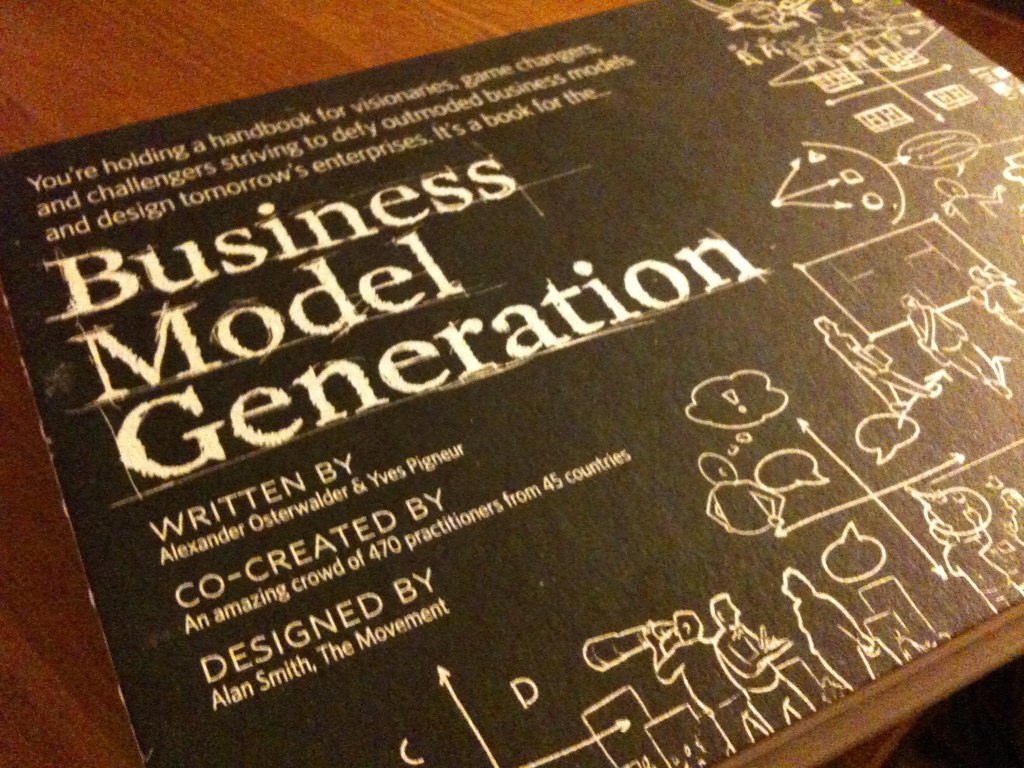In this detailed image, a single book is prominently displayed on a large, brown, wooden table, situated indoors. The book, almost perfectly centered, features a predominantly black cover adorned with intricate white drawings, including images of people using telescopes and various mathematical angles. The prominently displayed text on the book's cover reads: "You are holding a handbook for visionaries, game changers, and challengers striving to defy outdated business models and design tomorrow's enterprises." In large, white font, the title "Business Model Generation" stands out. The book is authored by Alexander Osterwalder and Yves Pigneur, co-created by an impressive crowd of 470 practitioners from 45 countries, and designed by Alan Smith of The Movement. The colors present in the image include shades of brown, black, white, off-white, and hints of yellow. Although the time of day is indeterminable, the setting appears distinctly like a table or countertop, suggesting an indoor location.